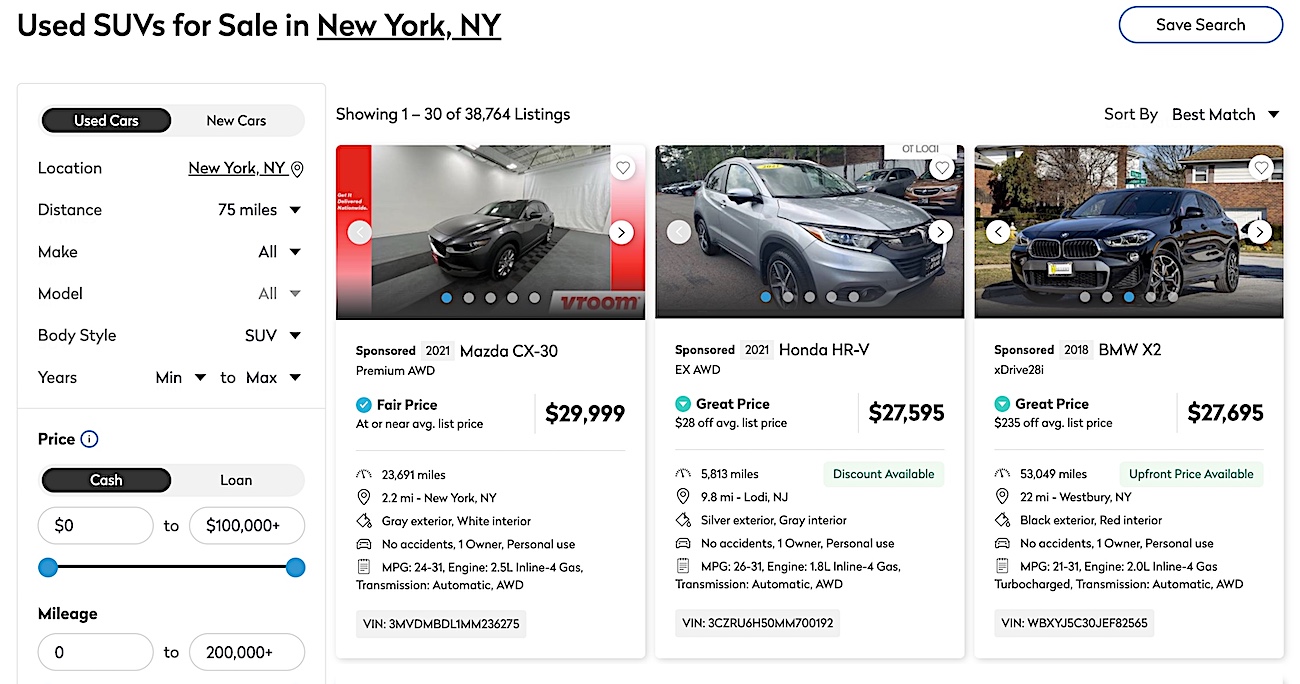**Detailed Caption:**

A selection of SUVs available for sale in New York, New York, encompassing both used and new vehicles. The listing features a total of 38,764 entries, with individual car details displayed as numbers 1 through 30. The inventory is offered within a 75-mile radius of New York, New York, and includes various makes, models, and price ranges. 

Highlighted in the list is a black 2021 Mazda CX-30 SUV with all-wheel drive. This vehicle is priced at $29,999 and has accumulated 23,691 miles. Its location is 2.2 miles from New York, New York. The Mazda CX-30 sports a gray exterior and a white interior, with a clean history of no accidents and being a personal use car with only one previous owner. 

Performance details include a fuel efficiency rating of 24 to 31 miles per gallon, powered by a 2.5-liter inline-4 gas engine paired with an automatic transmission. The vehicle identification number (VIN) for this Mazda CX-30 is 3MVDMB1MM236275.

The listing is identified as at or near the average market price and is sponsored by Vroom. The visual of the vehicle includes a red border on the left and right sides, and is marked by four gray dots and one blue dot.